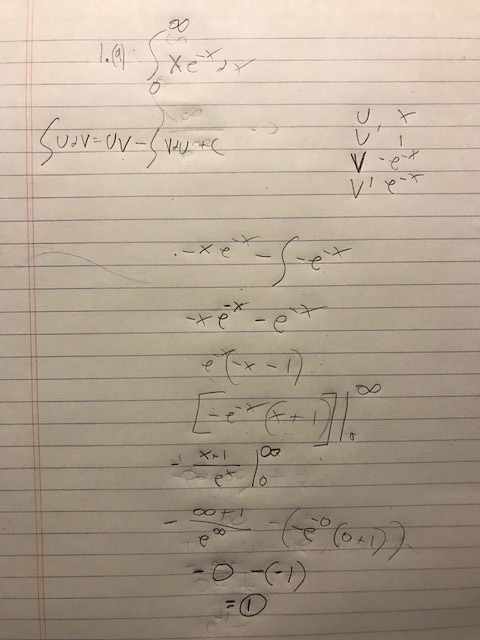The photograph depicts a classic sheet of lined white notebook paper featuring the characteristic thin double red lines marking the margin on the left side and evenly spaced blue lines running horizontally across the page. The page is densely filled from top to bottom with handwritten algebraic and calculus equations in pencil. The handwriting is somewhat sloppy, making deciphering the equations challenging.

Prominent among the mathematical notations is a squiggly bracket that resembles an elongated 'S'. There are several instances of expressions involving variables 'U' and 'V', such as "U something V" and "U of V or U+V". Some terms contain fractions and other complex notations indicative of higher mathematics, possibly calculus, which include symbols like 'U', 'X', 'U’', and '1'. Another noteworthy expression on the page involves terms like "V-E to the something power" and "V1E to the negative X".

Near the bottom of the sheet, a sequence of algebraic manipulations culminates in a notable line of text reading "negative 0 minus (negative 1)", which simplifies to "1", encircled emphatically. This elaborate and somewhat convoluted tableau of mathematical expressions suggests a detailed attempt at solving advanced mathematical problems, reflecting both the complexity of the subject matter and the personal struggle of the writer to organize their thoughts and computations clearly.